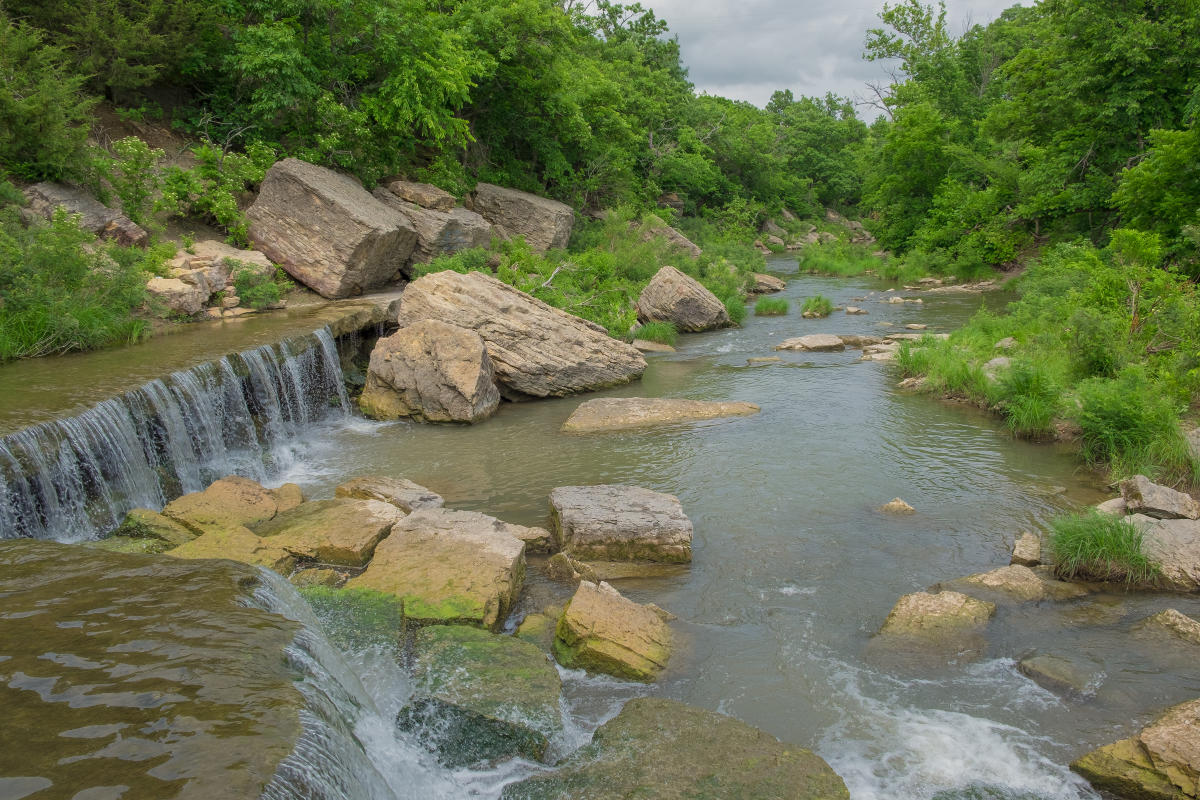The photograph captures a serene, albeit slightly murky, creek or river with notable natural features. Starting in the upper left, the water cascades over small, double waterfalls, splitting around a protruding stone and splashing down onto a bed of substantial, jagged rocks, which are predominantly brownish-gray, likely shale or sandstone in nature. The water continues its journey downstream through a narrow, rocky passage flanked by lush greenery. Tall, medium-growth trees with green leaves and luxuriant bushes hem in the scene, creating an enclosed, tranquil atmosphere perfect for solitude or a peaceful picnic. Despite hints of muddiness, the water retains a dark, greenish-gray clarity that allows glimpses of the creek bed. The sky above is overcast with gray clouds, adding to the secluded and calm ambiance of this natural spot.